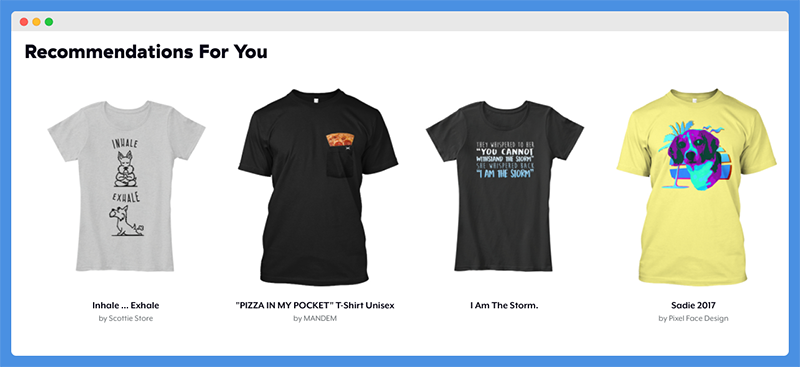This image is a screenshot from an unidentified source, outlined in dark blue. The background is white, with a light gray banner at the top. In the top left corner of the gray banner, there are three circles: a red circle, a yellow circle, and a green circle. Below this banner, in black lettering, it reads "Recommendations for you."

Displayed below this heading are photographs of four different short-sleeved shirts:

1. The first shirt is white and features an image of a dog doing yoga. At the top, it says "Inhale," with the dog sitting calmly with its paws pressed together in front of its chest. Below, it says "Exhale," showing the dog in a Downward Dog pose with a humorous fart cloud coming from its rear. The text "Inhale Exhale" is spelled "Inhale Exhale" and the design name "Scott" is spelled "SC OTT ie."

2. The second shirt is black with a pocket on the right side. Above the pocket, there is an image that makes it look as though a piece of pepperoni pizza is sticking out of the pocket. Below the image, the text reads "Pizza in my Pocket T-Shirt" and indicates that it is a unisex shirt by "Mandem," spelled "mand EM."

3. The third shirt is also black. It has the text "They whispered to me, 'You cannot withstand the storm.' She whispered back, 'I am the storm.'" underneath, the text simply repeats, "I am the storm."

4. The fourth shirt is yellow with an 80s style print featuring a beagle looking at the viewer. Behind the dog, there is a palm tree and a lined shape. Below the image, the text reads "Sadie 2017" by "Pixel Face Design."